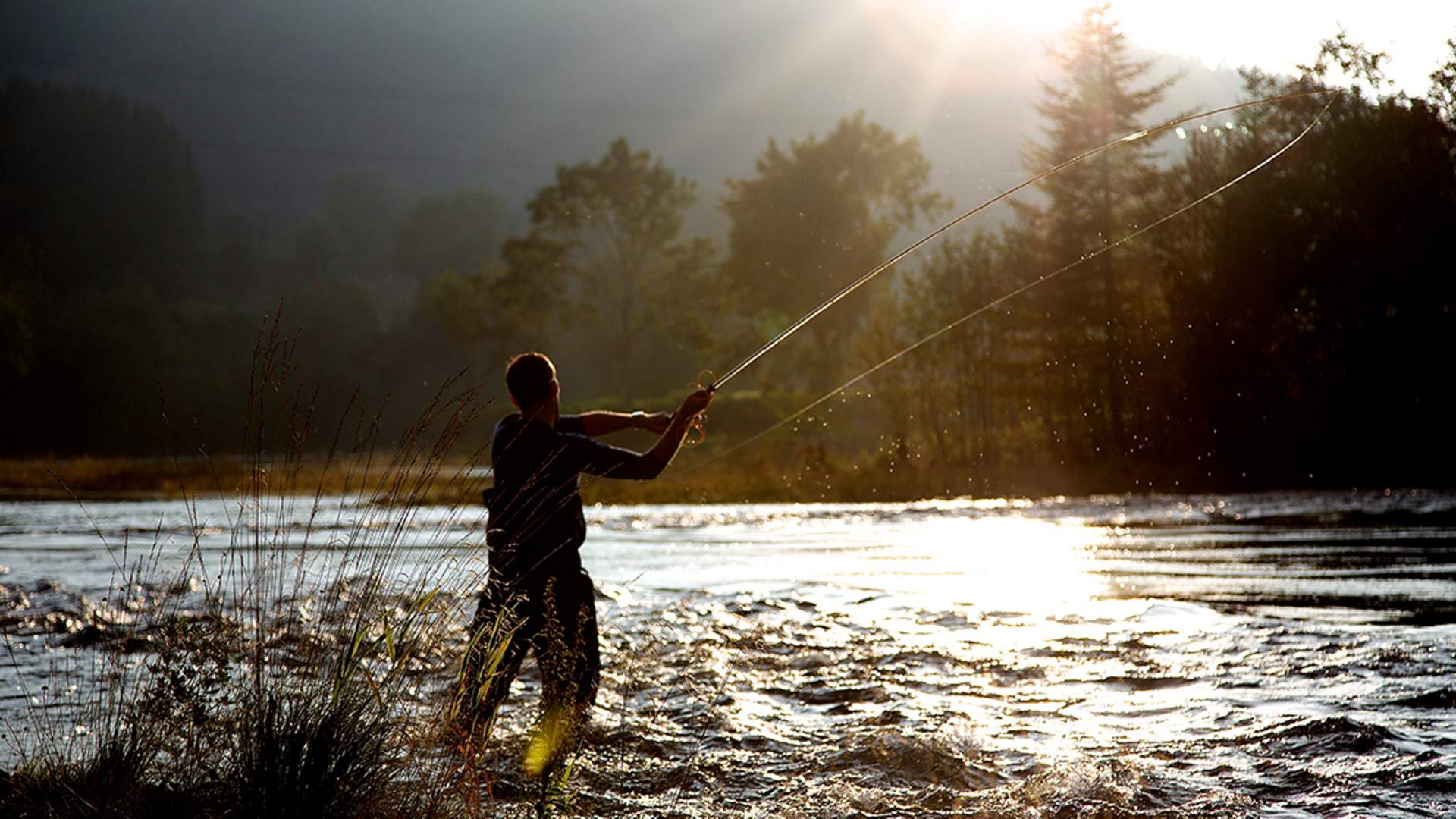In this detailed photograph, a man is fishing in a river, which occupies the bottom third of the frame. The river surface is choppy, with a spectrum of colors from a grayish-blue on the left, transitioning to black on the right, and a brilliant white-golden glow in the center where the sun reflects off the water. The fisherman stands knee-deep in the water, slightly right of a large silhouetted tuft of grass in the bottom left corner. He wears baggy black wader pants and a black short-sleeved shirt, his posture showing him casting his fishing pole back in a gentle arc. His short hair emits a reddish-brown glow under the sunlight. The scene is dramatically lit with the sun bursting from the top right, creating sun rays and Jacob's Ladders that beam downwards across the image. In the distance, a flat terrain with brownish grass and a variety of pine and deciduous trees recedes towards the horizon, where a dark outline of a hill or mountain range is visible, enhancing the tranquil beauty of this natural setting.